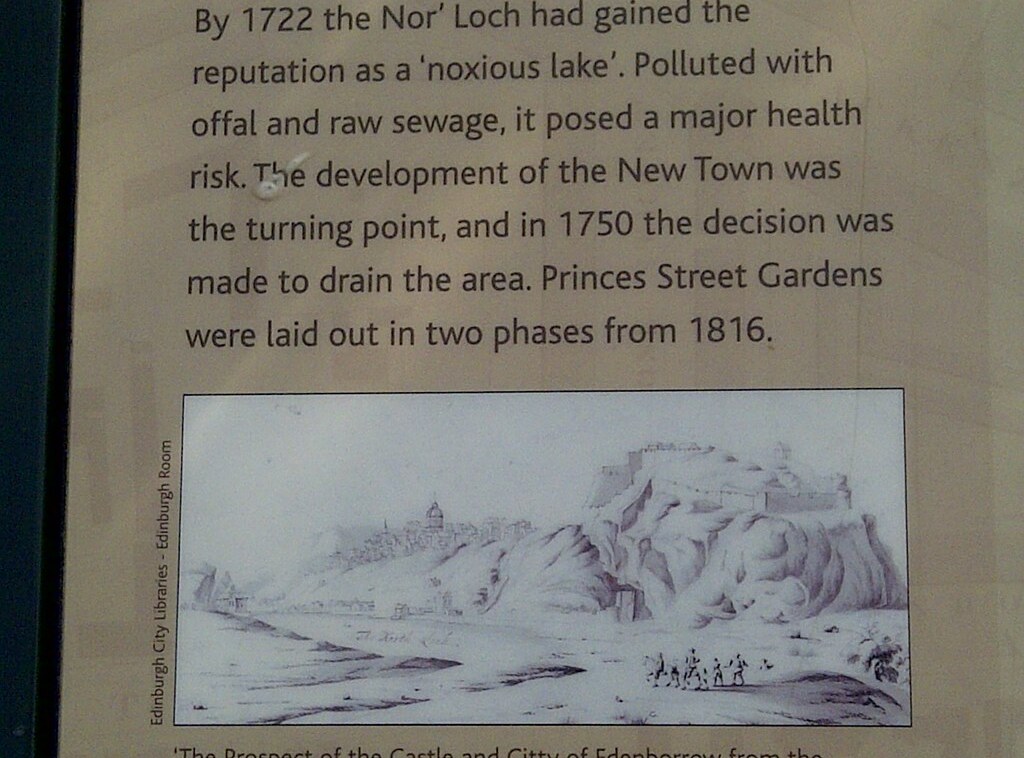The image appears to be a framed historical signage or poster, likely displayed at a historical site. The left side of the poster is marked by a prominent black line, suggesting a frame border. The text on the poster, set against a light brown background with dark brown lettering, reads: “By 1722, the Norlock had gained the reputation as a noxious lake, polluted with offal and raw sewage. It posed a major health risk. The development of the new town was the turning point, and in 1750 the decision was made to drain the area. Princess Street Gardens were laid out in two phases from 1816.” Below the text, there's an old, grainy black and white illustration. This depicts people crossing a landscape with a large hill or mountain in the background, a village, and possibly a fort or castle on the left side. The illustration is labeled “Edinburgh City Libraries, Edinburgh Room.”